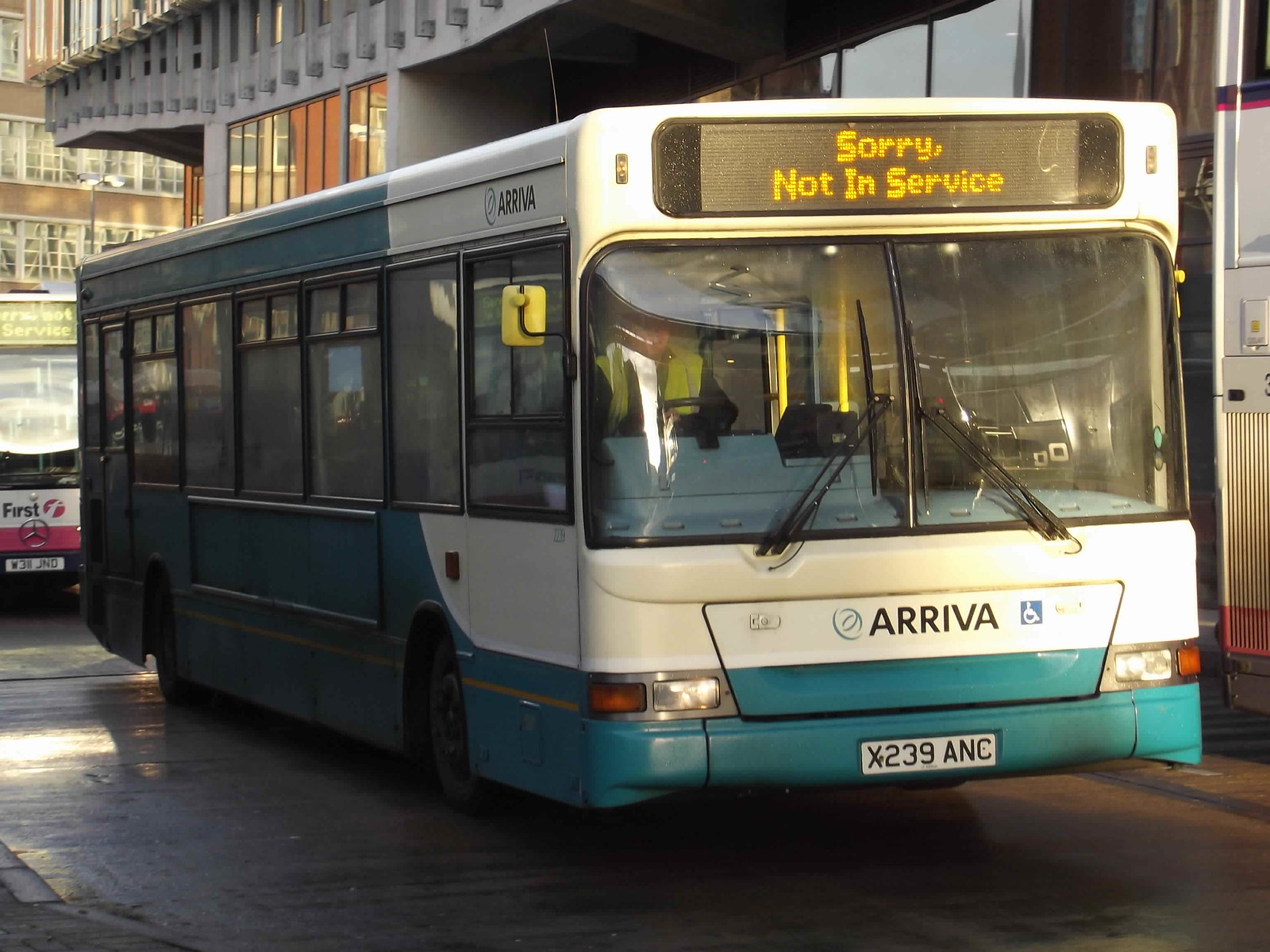This photograph captures a scene in an urban setting featuring two parked city buses in front of modern buildings. The primary bus in the foreground is predominantly white with a blue bottom bumper extending along its side. It displays the Arriva logo on both the front and the upper right side panel. The license plate reads X2398NC, suggesting a European location. Notably, an LED placard at the top front of the bus states "Sorry, Not in Service" in yellow text against a black background. 

The bus exhibits a blocky and square-like frame and has a mixture of white and light green colors visible on its front and side, including six windows along its side. Additional features include black windshield wipers centrally positioned on the front windshield and a blue square handicap logo with a white silhouette of a person in a wheelchair.

Behind this bus, another bus can be seen, identifiable by its white and pink coloration and a similar "Sorry, Not in Service" sign. Both vehicles are parked on a black asphalt street adjacent to what seems to be a clean, cement building with numerous windows, typical of urban architecture. No people are seen inside the buses or milling about, hinting that this may not be a busy area, and there is no clear indication of a bus or train terminal nearby.